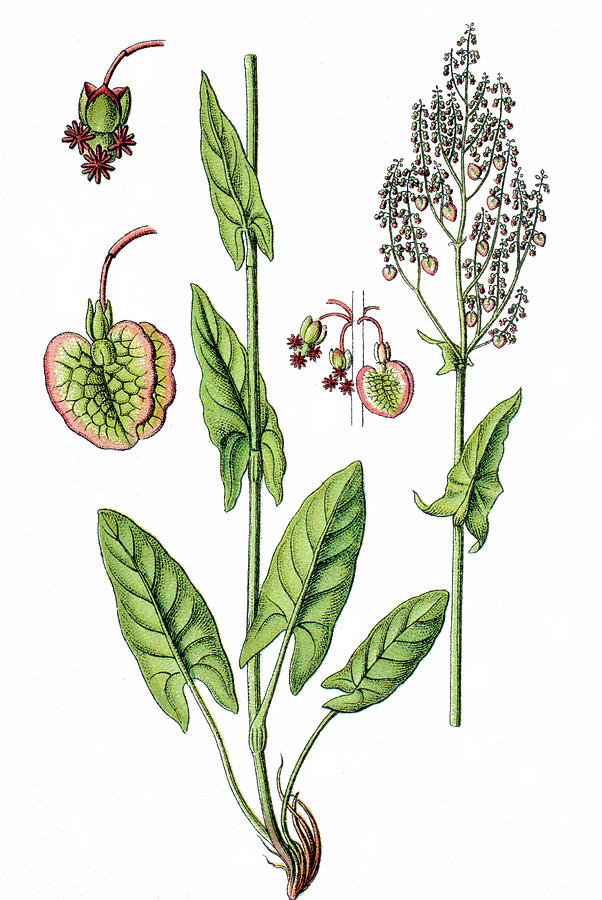The image resembles an illustration from a botanical textbook, featuring detailed graphic depictions of a plant against an all-white background. At the top left, a close-up of the plant reveals reddish-green fruits still attached to a branch, highlighted in an animated style reminiscent of botanical drawings. On the far right, the plant is shown in its entirety, displaying a slender, wavy stem with multiple arrowhead-shaped leaves and small, star-shaped flowers or fruits at the tips, blending green and red hues. In the center, another close-up focuses on the plant's wavy, pointed leaves and the emerging seeds. The image emphasizes the plant's intricate details without any accompanying text, offering a vibrant and educational look at its structure.